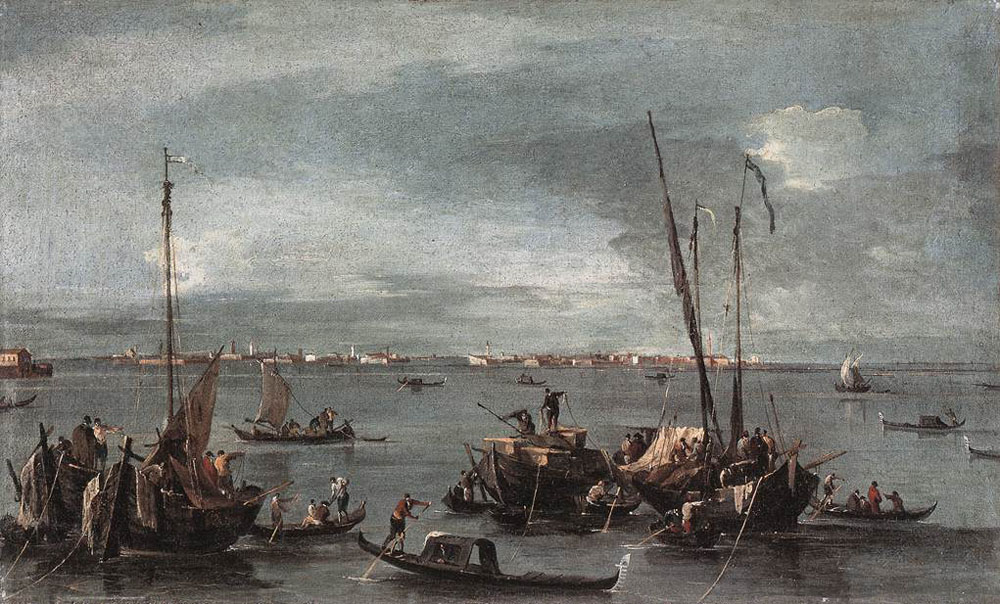This detailed painting captures a serene seascape within a harbor, rendered in a horizontally aligned rectangular format. The sky at the top is overcast, blending soft gray, blue, and tan tones with puffy cloud formations suggesting an impending storm. Below the sky, the distant horizon features a cityscape of brown, tan, and white buildings, with outlines of houses and cottages peeking through.

In the middle ground, numerous boats populate the calm, dark gray waters, which are speckled with white spots. The vessels range from small kayaks and gondolas to larger sailboats and ships. Many of the boats have their sails retracted, indicating that they are docked or anchored. The sailors aboard are depicted standing, engaged in various tasks, some rowing gently with oars. 

Central to the composition is a man wearing red and black, standing on a tiny, almost kayak-like boat with a tent over it, navigating with his oar in the water. The overall scene conveys a bustling yet tranquil atmosphere, with intricate details highlighting the labor and leisure intertwined in this picturesque harbor.